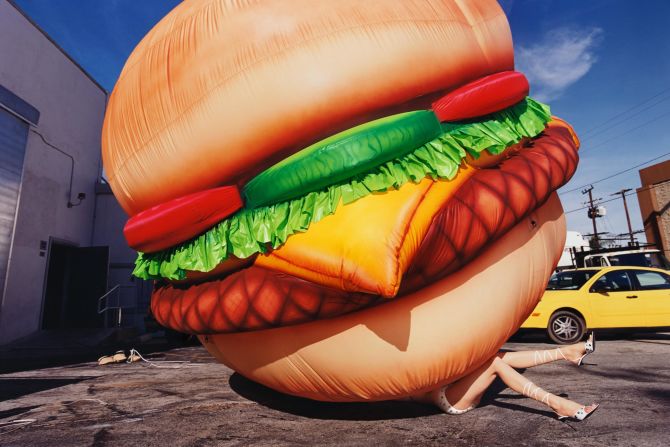This surreal, cartoon-like image depicts an oversized cheeseburger, resembling an inflatable costume, seemingly fallen onto or crushing a woman dressed in a bikini bottom and high heels with laced-up shoes reaching mid-calf. The burger, nearly 10 feet in size, dwarfs everything around it, including a nearby yellow car with black mag wheels to its right. The cheeseburger is detailed with layers of cheese, lettuce, pickles, and tomatoes on a brown bun, emphasizing its exaggerated proportions. The scene is set in what appears to be a parking lot, with a whitish-gray building featuring a black, open door accessible by a few steps on the left. The blue sky in the background, lightly dotted with clouds, contrasts with the almost industrial setting and amplifies the bizarre, playful nature of the composition.